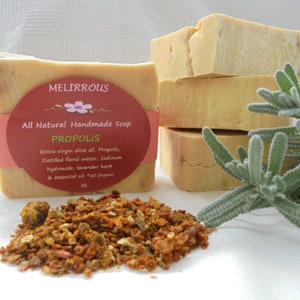This promotional image for Maliris All Natural Handmade Soap showcases a clean, minimalist aesthetic with a white table and background. Front and center, a bar of handmade soap with an imperfect, beige appearance features a notable red label. The label, predominantly dark pink, reads "Maliris All Natural Handmade Soap, Propolis," followed by smaller, unreadable text. Adjacent to the soap is a small, colorful pile of chopped ingredients, including orange, tan, and beige pieces that resemble herbs or potpourri. To the right, a stack of three similar soaps is highlighted, with the top bar notably cracked on the side. A sprig of cactus contributes a touch of green to the composition, enhancing the natural theme of the advertisement.